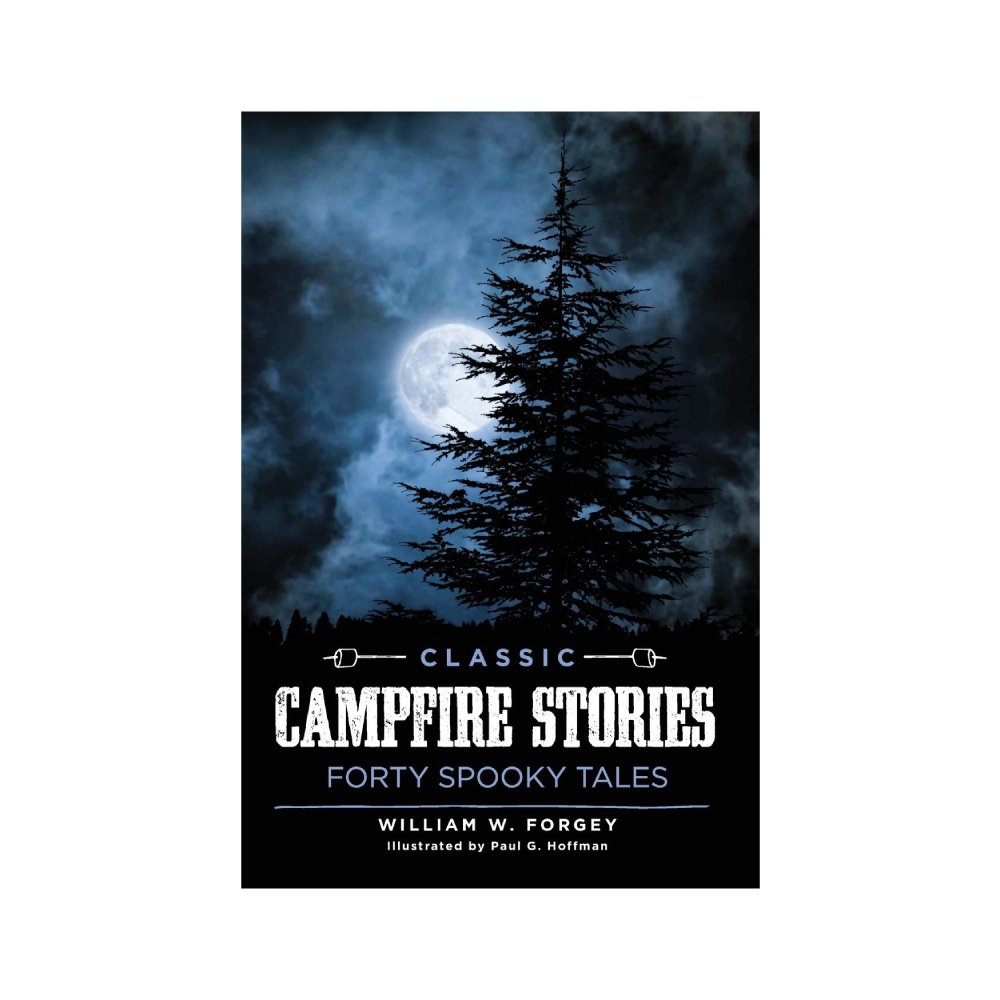The image is a detailed book cover designed to evoke a spooky, nighttime atmosphere. Dominating the upper portion is a photograph of a lone evergreen tree set against a foggy night sky, where the tree appears as a dark silhouette due to the full moon shining brightly behind it. Ethereal clouds, illuminated by the moon, add an eerie, ghostly effect to the scene. The lower third of the cover is a black background with text. At the bottom, blue text reads "Classic," flanked by clipart of marshmallow sticks on each side. Just below, in larger bold white letters, it says "CAMPFIRE STORIES." Beneath that, in smaller blue text, it states "40 Spooky Tales," and below that, in white, it lists the author, "William W. Forgey," and the illustrator, "Paul G. Hoffman."